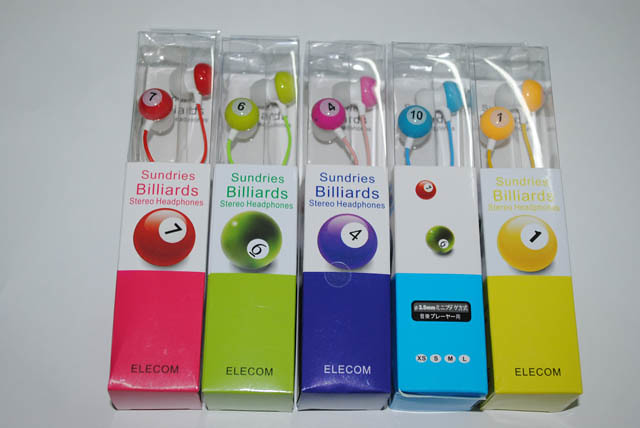This photograph presents five distinct packages of earbuds arranged horizontally against a light gray background. Each rectangular package features clear plastic through which the earbuds are visible, with the top part adorned by colored cardboard labels that correspond with the color of the earbuds. 

From left to right, the colors and details are as follows:

1. **Red Packaging**: This pack showcases red earbuds labeled with a red billiard ball bearing the number seven. The brand name “Sundries Billiards Stereo Headphones” and the manufacturer name “Elecom” are marked on the packaging.
   
2. **Yellow/Green Packaging**: This pack has yellow/green earbuds paired with a yellow billiard ball labeled with the number six. Similar to other packages, it includes the brand name “Sundries Billiards Stereo Headphones” and “Elecom.”
   
3. **Purple Packaging**: Although the earbuds inside are pink, the package is purple with a purple billiard ball marked with the number four. The brand and manufacturer names are present, but the word “Elecom” is written in white instead of black.
   
4. **Light Blue Packaging**: The light blue earbuds are labeled with a light blue billiard ball marked with the number ten. This package has additional black rectangles with Asian writing and does not have the word “Elecom” written on it.
   
5. **Yellow Packaging**: This package carries yellow earbuds and a yellow billiard ball with the number one. Consistently, it includes the “Sundries Billiards Stereo Headphones” and “Elecom” designations.

Each package integrates a circular billiard ball image with its respective number inside a white circle, matching the conventional billiards theme and adding a playful, distinctive character to the earbuds and their branding.